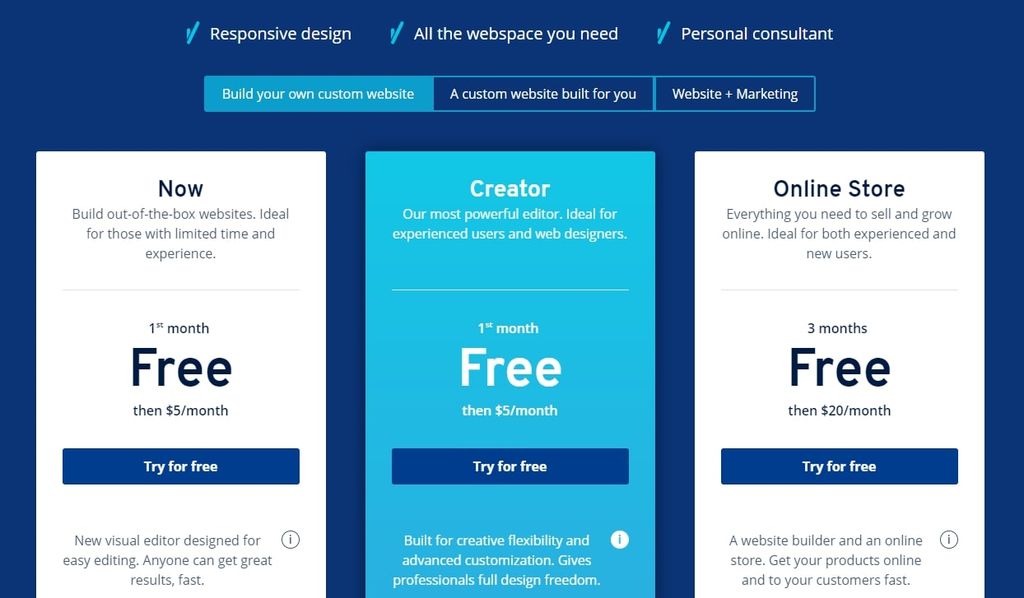**Detailed Caption:**

The image is a cropped screenshot of a website builder interface with a blue background. At the top, three key features are listed centrally, each accompanied by a blue check mark. From left to right, the first feature is "Responsive Design". The second feature is "All the Web Space You Need". Lastly, the third feature is "Personal Consultant".

Below these statements, there are three highlighted options, each in a box. The first option, which is highlighted in blue with white text, reads "Build Your Own Custom Website". The second option in the middle is "A Custom Website Built for You". The third option on the right states "Website and Marketing".

The first option, "Build Your Own Custom Website", is selected. Beneath these options are three horizontally arranged rectangles outlining different service tiers:

1. **Left Rectangle**:  
   - **Background**: White  
   - **Title**: "Now" in large letters  
   - **Description**: "Build out-of-the-box websites ideal for those with limited time and experiences."  
   - **Pricing**: "First month free, then $5 a month"  
   - **Button**: "Try for Free"

2. **Middle Rectangle**:  
   - **Background**: Light blue  
   - **Title**: "Creator" in large white font  
   - **Description**: "Our most powerful editor ideal for the experienced users and web designers."  
   - **Pricing**: "First month free, then $5 a month"  
   - **Button**: "Try for Free"

3. **Right Rectangle**:  
   - **Background**: White  
   - **Title**: "Online Store"  
   - **Description**: "Everything you need to sell and grow online, ideal for both experienced and new users."  
   - **Pricing**: "Three months free, then $20 a month"  
   - **Button**: "Try for Free"